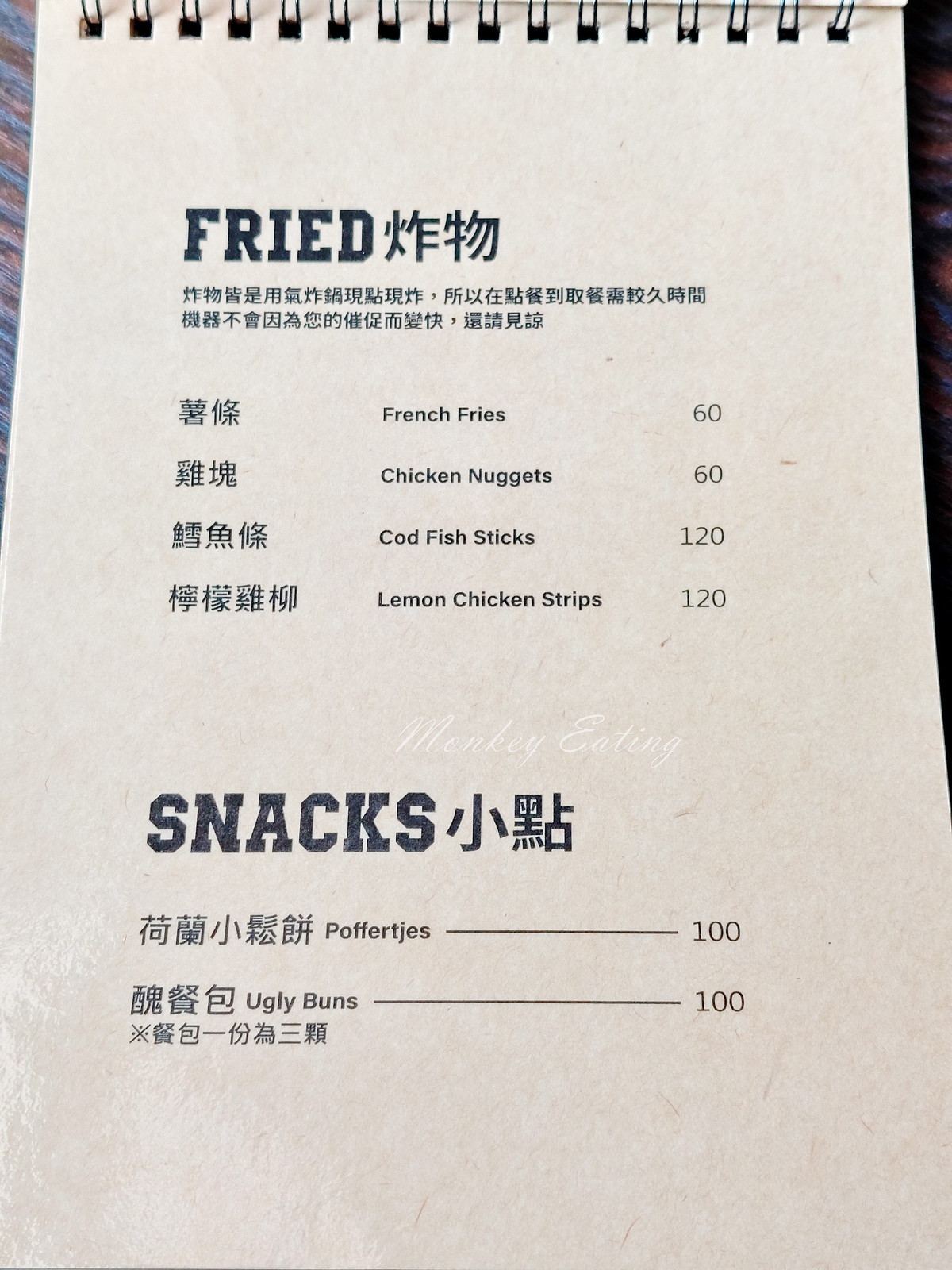The image captures a unique menu presented in a wire-bound, notebook-style format with pages designed to flip over like a steno pad. The page visible to us is written in either Chinese or Japanese and features clearly listed prices. The first section of the menu is titled "Fried" and includes four choices: french fries, chicken nuggets, cod fish sticks, and lemon chicken strips. Following that, there's a "Snacks" section offering a few intriguing options including "pofert cheese" or "pofert jays" and an item intriguingly named "ugly buns". This is just one of the pages from the menu, suggesting that additional options are available on subsequent pages.